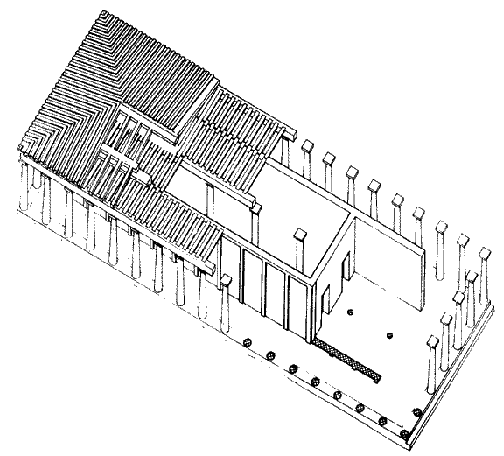This black and white pencil or pen architectural drawing depicts a rectangular building viewed from an aerial, diagonal perspective, running from the top left to the bottom right of the image. The structure is outlined in black against a plain white background, exhibiting various stages of architectural development. On the left side, you can see the initial placement of a few columns, which progressively increase towards the right, revealing the construction stages with more columns, partial walls, and doorways emerging. The building seems to be a long hall with its roof supported by columns all around the perimeter. Inside, there is another structure with walls and doors, indicating a more complex internal design. The drawing is meticulous yet simple, devoid of any text, making it a pure representation of an architectural concept in its developmental stages.